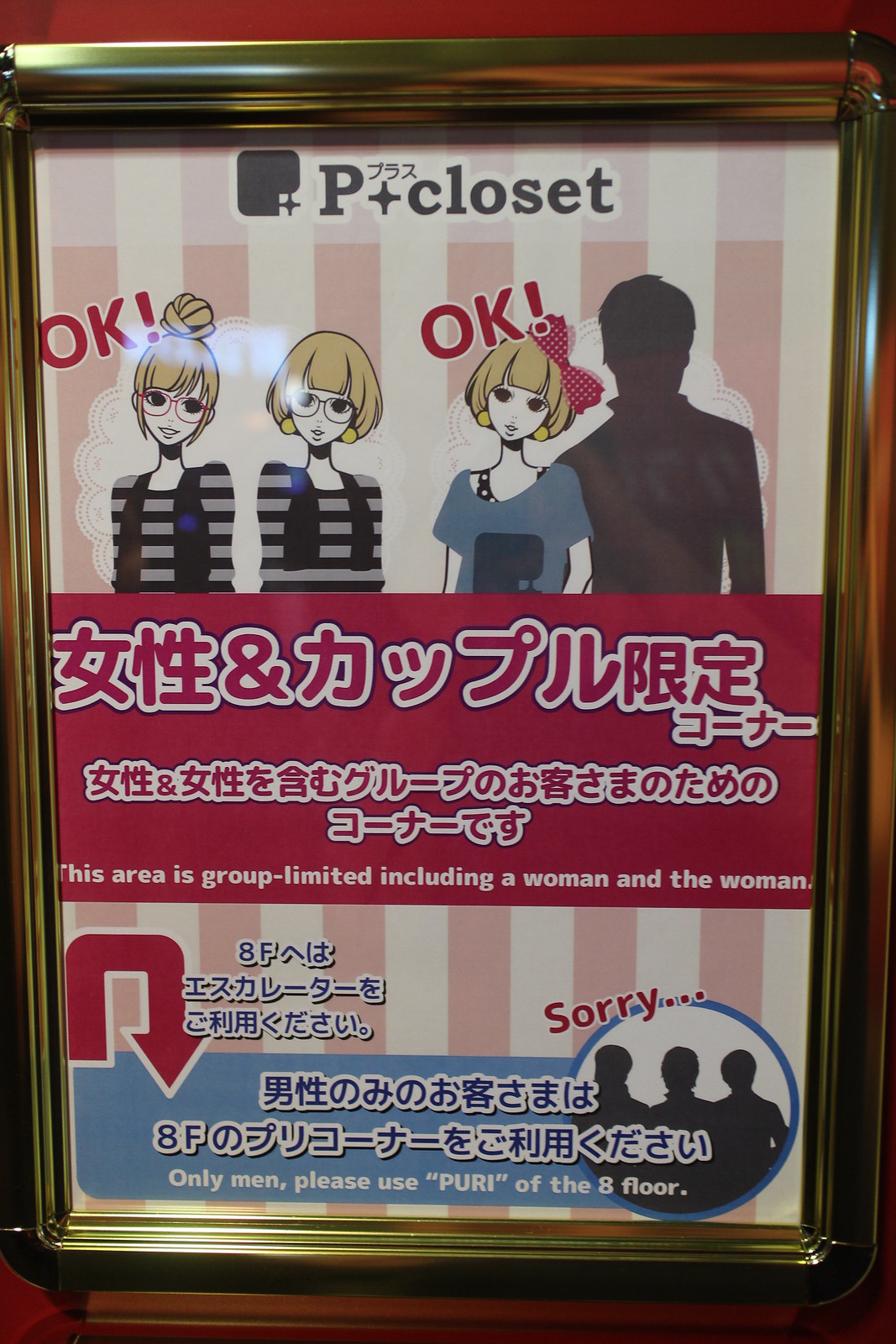The image depicts a plaque with a gold or brass frame and features predominantly Asian writing, likely Chinese or Japanese. Central to the plaque are four cartoonish yet semi-realistic characters: three young women and a silhouette of a man. There are two instances of the word "okay!" with exclamation points, one above the leftmost woman and one above the rightmost woman. Sparse English text on the plaque reads, "this area is group limited, including a woman and the woman," and below, "ONLY MEN, PLEASE USE PURI OF THE EIGHTH FLOOR," in bold capitals. The background colors are mostly faded, lending an aged or vintage feel to the sign. The plaque also bears the title "P Plus Closet" at the top. The surrounding context is unclear due to the close-up nature of the image, but there is a faint reddish hue at the bottom of the sign, possibly indicating some sort of restriction or warning.